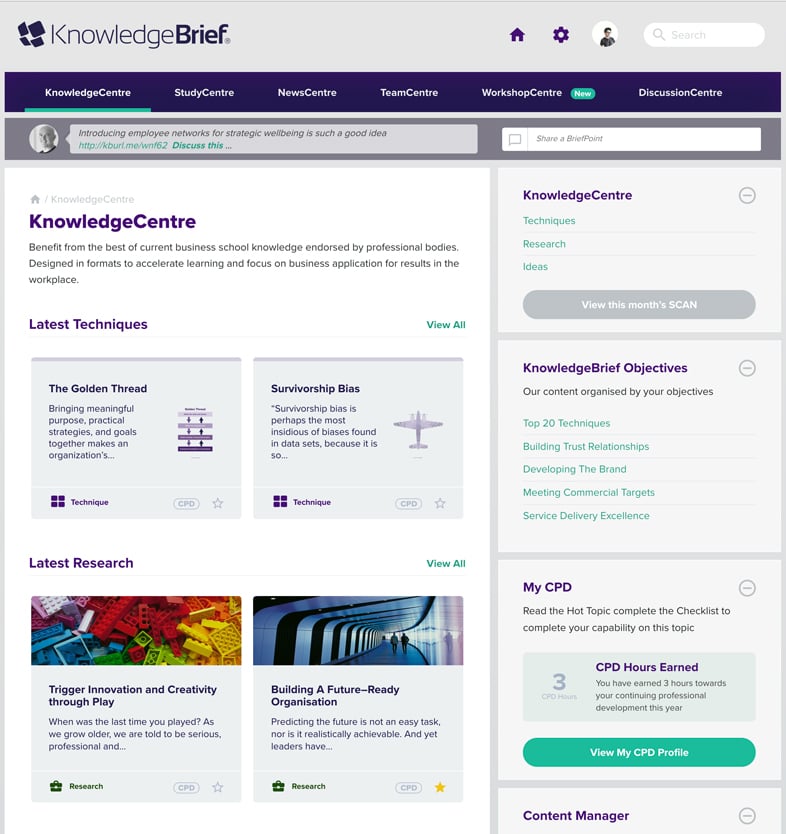This image is a screenshot of a website's webpage, designed with a clean and functional layout. 

At the very top, there is a grayish navigation bar running horizontally across the page. On the left side of this bar, the text "Knowledge Brief" is displayed, with "Brief" emphasized in bold letters. Accompanying this text on the left are several square icons, while on the right side of the bar are icons for ‘Home’, ‘Settings’, a user profile icon enclosed in a white circle, and a search bar.

Directly below this, there is a purple menu bar with white text. This menu provides various options such as "Knowledge Centre," "Study Centre," "News Centre," "Team Centre," "Workshop Centre" (noted as 'new'), and "Discussion Centre." The word "Centre" is spelled with the British variant "-tre" in all instances. Below this menu, a prominent pull quote from a bald gentleman states, "Introducing employee networks for strategic well-being is such a good idea."

Further down, a search bar is present with the prompt “Share a brief,” suggesting interactivity and user contribution. Below this, another heading in purple reads "Knowledge Centre." The section emphasizes benefiting from the latest business school knowledge, endorsed by professional bodies, and designed to accelerate learning and practical application in the workplace.

Beneath it are two description boxes in gray. The box on the left is titled "The Golden Thread," which hints at the importance of aligning meaningful purpose with practical strategies and goals for organizational success. The text cuts off with an ellipsis. The box on the right discusses "Survivorship Bias," indicating it as a critical but often overlooked bias in data sets, also ending with an ellipsis.

This layout suggests a comprehensive resource center aimed at enhancing business knowledge and practical application.